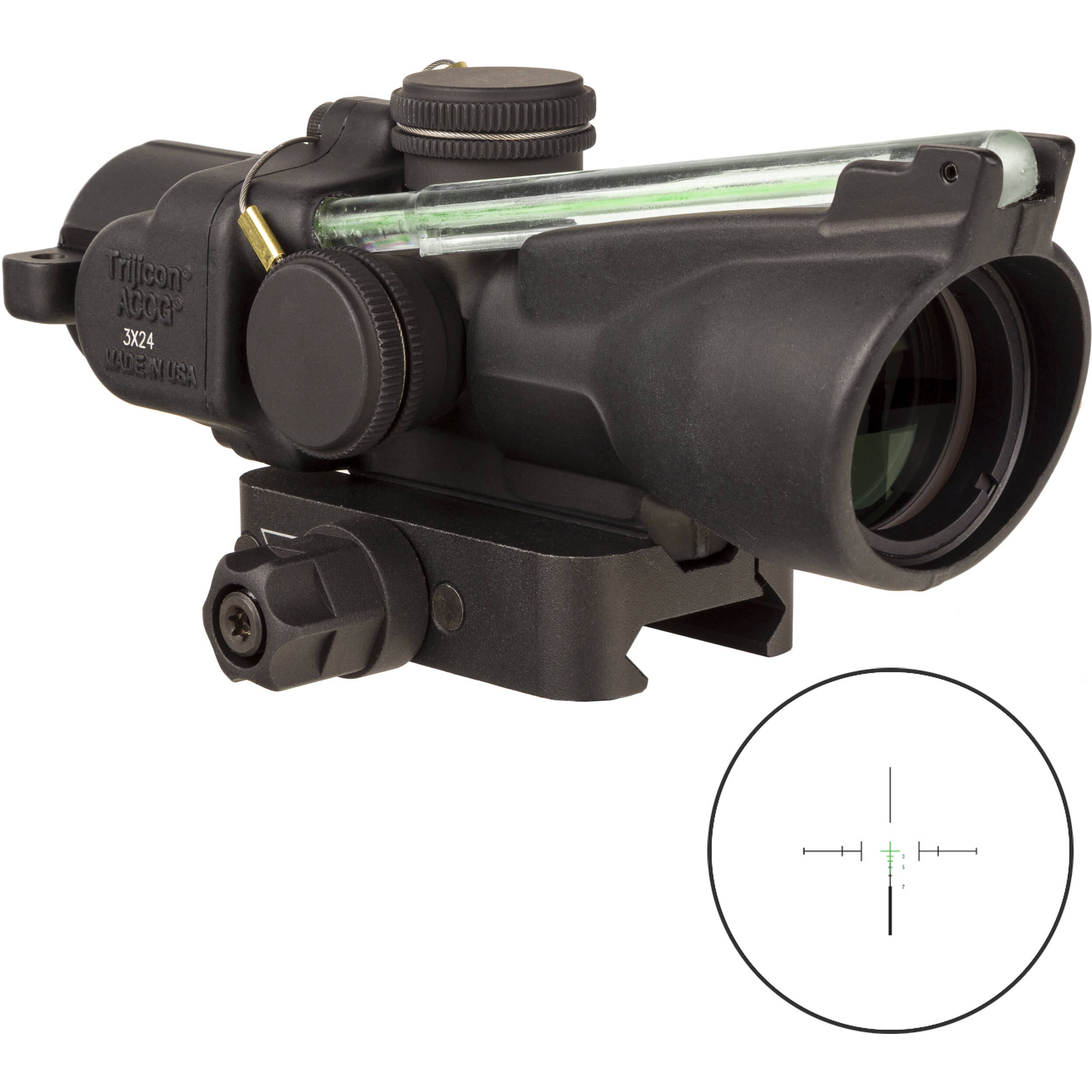This image showcases a high-quality product shot of a Trijicon ACCG scope, prominently centered and designed for precision viewing. The scope is primarily black with a slender silver metal rod along its top, emphasizing its sleek construction. It features a cylindrical body that flares towards the glass lens end for better field view. There are three dials on the scope: two flat circular ones integrated into the main body and a third hexagonal dial, likely for fine adjustments. For mounting, it includes a sliding attachment mechanism with a screw and nuts at the bottom, compatible with tripods.

Text beneath the scope states "Trijicon ACCG" in black, "3x24" in white, followed by "Made in USA" in black, indicating its magnification and manufacturing details. An inset near the bottom right corner displays a reticle—a crosshair diagram featuring a green cross within a black circle—illustrating what the viewer would see through the scope, which may even hint at night vision capabilities. This well-detailed image gives a comprehensive look at the Trijicon ACCG scope, highlighting its advanced design and features for potential users.